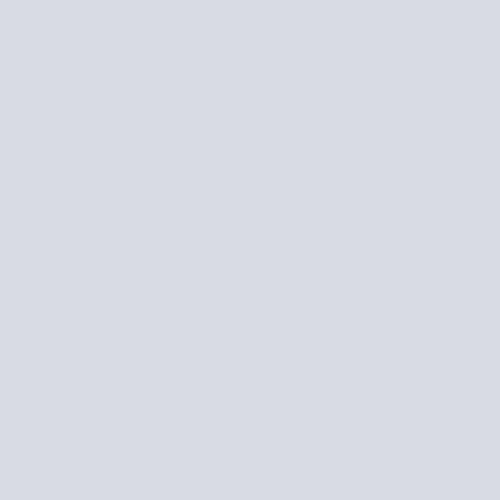The image features a large, well-defined square with smooth borders and a uniform dove-gray color. There are no other visual elements, such as text or images, within the square. The square lacks any pixelation or blurring, and the color is consistently even without any noticeable shadowing.